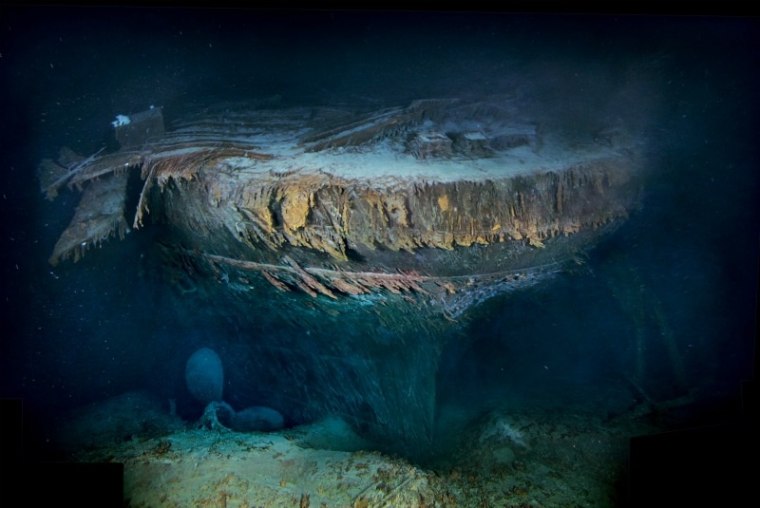The image depicts the haunting remains of a sunken ship, resting solemnly on the ocean floor. The vessel, in a severe state of decay, is almost completely disintegrated and covered in a thick layer of brown, shipwreck-esque material. The aft port section is discernible, featuring a propeller and what might be the rudder. The scene is partially illuminated, revealing the rotted and collapsed structures on the main deck and wooden panels amidst debris. There are scattered bubbles and white silty particles hovering around, contributing to the eerie atmosphere. The dark, ocean blue hue borders the image, emphasizing the underwater setting, and scattered boulders and rocks can be seen in the background. The surrounding darkness makes the submerged ship blend into the seabed, creating a stark contrast with the selectively highlighted areas, lending an otherworldly quality to this ghostly underwater tableau.